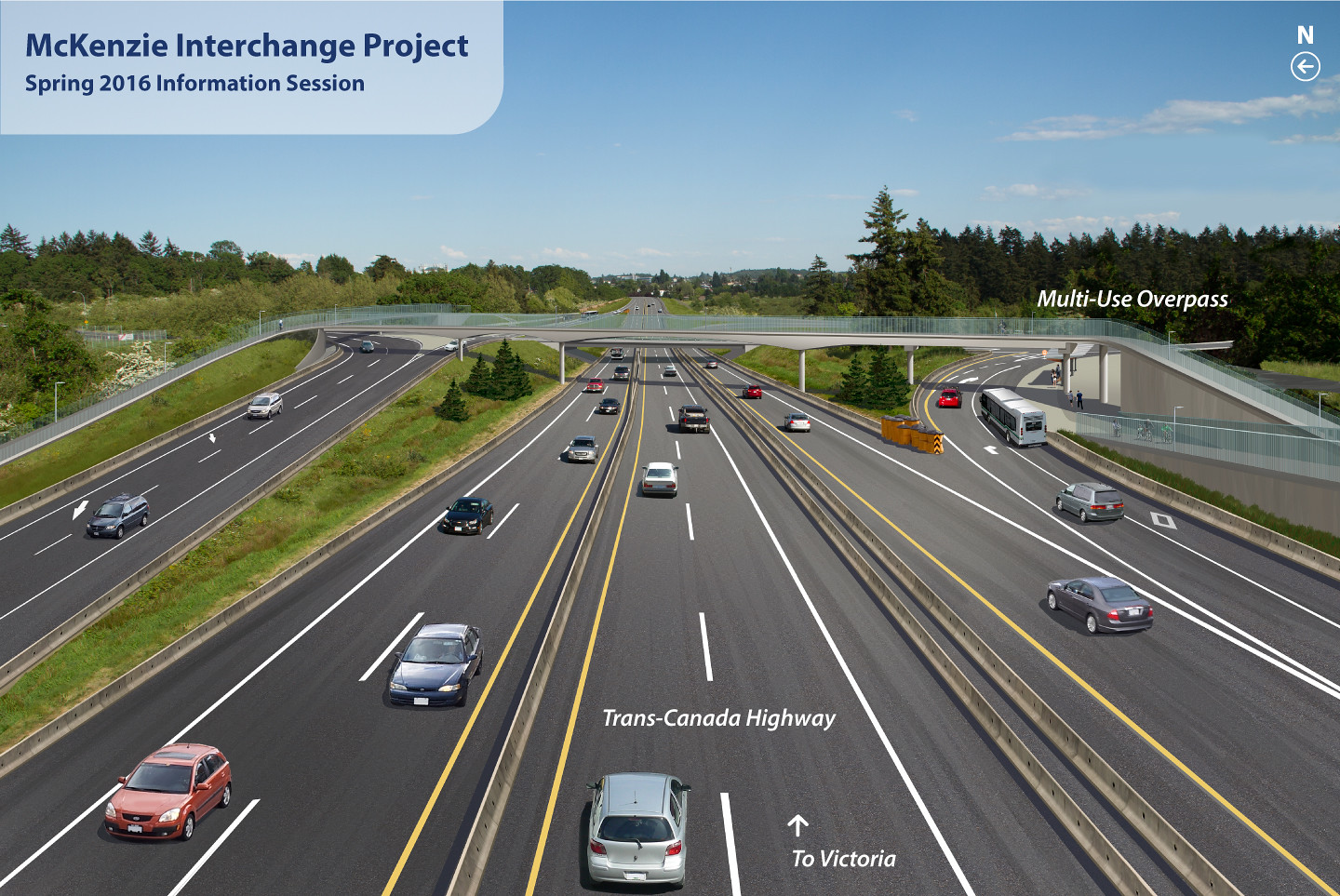The image presents a detailed rendering of the McKenzie Interchange Project, as showcased during the Spring 2016 Information Session. In the top-left corner, a light blue rectangle contains the text "McKenzie Interchange Project" with "Spring 2016 Information Session" beneath it. The upper third of the image features a blue sky with scattered clouds, against a horizon lined with tall, green leafy trees and grassy expanses. Beneath this horizon, the intricate highway system is depicted, with four divided highway sections that include multiple lanes of traffic. 

The two leftmost sections are curved, converging into the middle lanes that continue towards the background, while the far-right section features another turn extending out of view. The overpass spans from the left to the right side of the image, including a multi-use section for pedestrians. Text labels within the rendering identify specific roads, including "Trans-Canada Highway to Victoria," and the "Motius Overpass." Various vehicles, such as cars and buses, are visible on the highway. In the distance, buildings rise faintly on the horizon, adding to the depth and complexity of the depicted infrastructure.